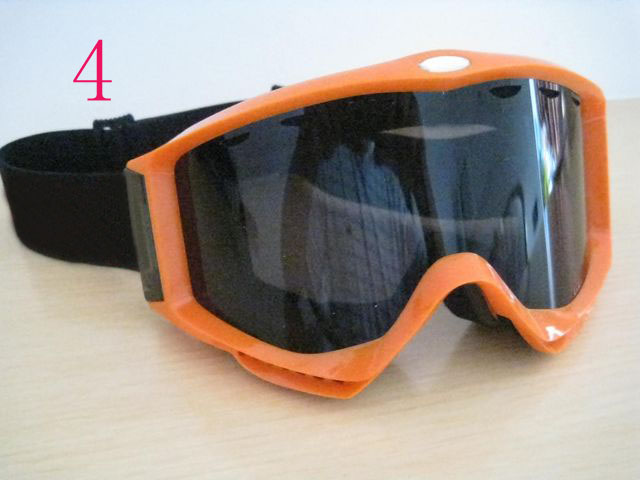The image showcases a pair of safety goggles with an orange frame around a single, large, dark gray-tinted lens. These goggles are positioned on a light, oak-colored wooden table, with a white wall serving as the background. The goggles are angled slightly towards the bottom right corner, giving a clear view of the thick, black elastic headband behind them. A prominent red number "4" is displayed in the upper left corner of the image. The lenses are highly reflective, capturing a distorted reflection of the photographer, who is identifiable by a white button-down shirt with a checkered pattern, holding what appears to be a cell phone. The lenses, shaped to fit snugly around the face with a noticeable nose indent and vent holes underneath the eye sockets, also feature a white dot at the center top, adding to the detailed design.